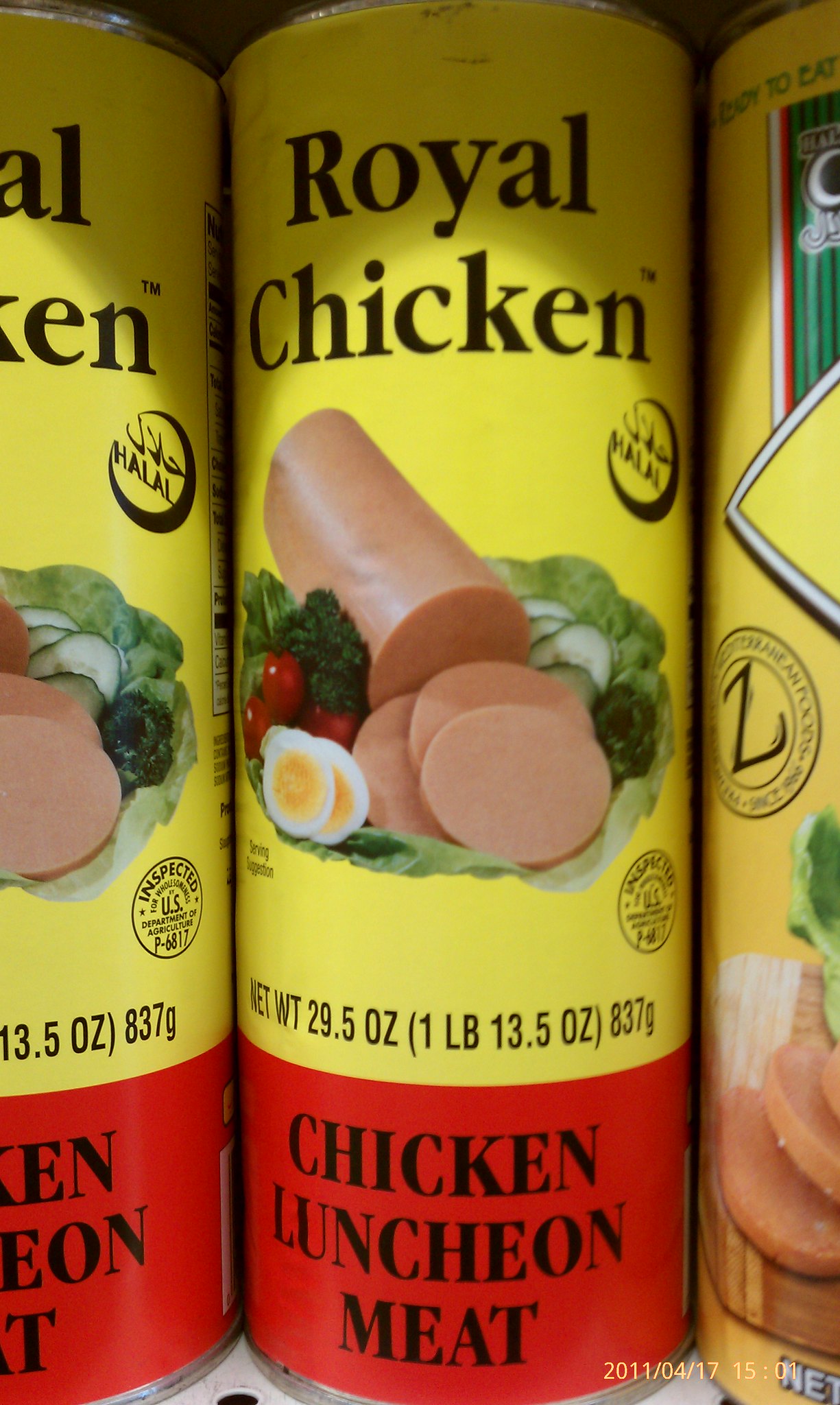The image captures a color photograph of several cans of canned luncheon meat, prominently featuring "Royal Chicken" chicken luncheon meat. The cans have a predominantly yellow label with a red horizontal section at the bottom. The front label of the central can displays the brand name "Royal Chicken" along with a Halal stamp and a U.S. inspector logo, indicating that the meat has been inspected. Below the brand name, the label states "Chicken Luncheon Meat" along with the net weight of 29.5 ounces (1 pound 13.5 ounces or 837 grams). The can showcases an image of the contents, presenting a beige to light brown, sausage-like chicken meat sliced and arranged on a bed of lettuce. The display includes accompanying garnishes such as cucumber slices, tomatoes, radishes, and a couple of hard-boiled eggs. The photograph, likely taken in a store, shows this central can flanked by another can of the same brand to its left and a different brand to its right, suggesting a retail setting with similar products shelved side by side. The photo also has a timestamp of 2-11-04-17-15-01 at the bottom.